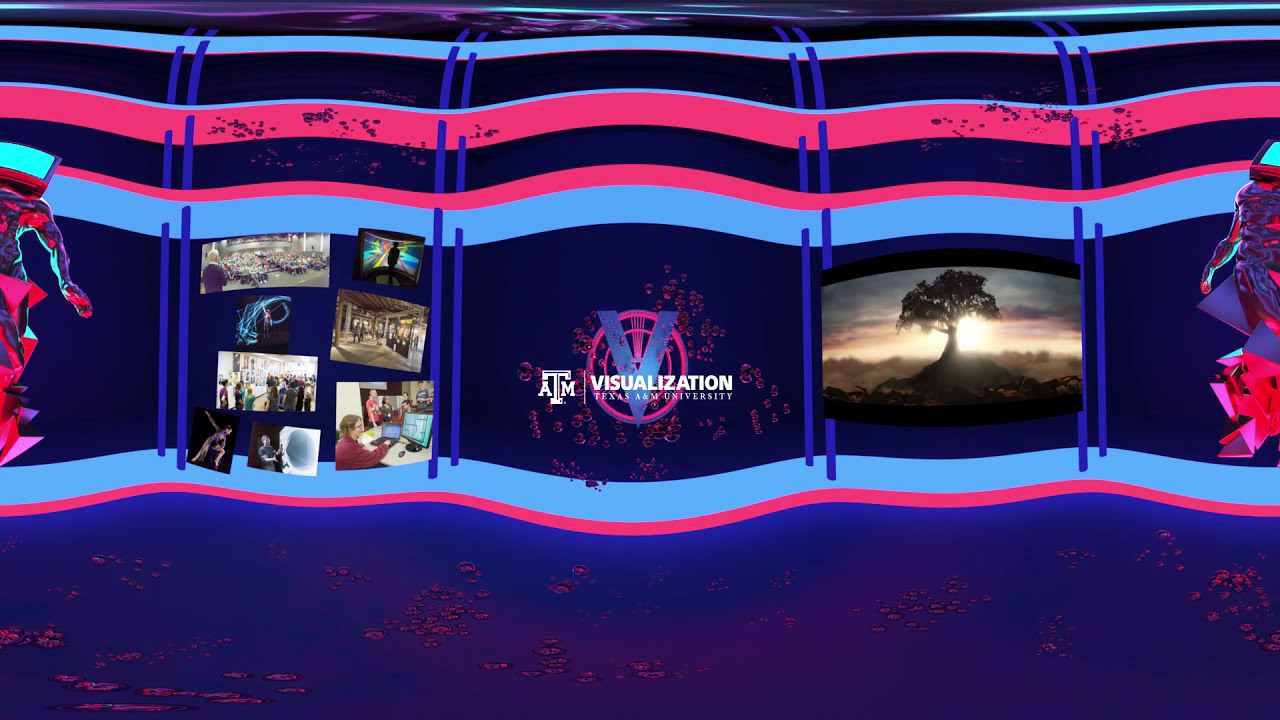The rectangular image, roughly six inches wide by three inches high, features a complex, surreal scene dominated by a wavy, horizontal band of navy blue with a light blue border. This undulating band resembles a distorted ladder, expanding and narrowing as it stretches across the image. Each narrowing point contains two vertical blue stripes, creating distinct sections. The most central section showcases a large blue "V" with purple rings behind it and white text reading "Texas A&M University Visualization." To the right, an image of a silhouetted tree against a sunset, evocative of scenes from the movie Avatar, adds a touch of natural beauty. To the left, a collage of diverse photographs depicts a statue, people engaged in various activities such as dancing and speaking, and a man at a computer. The bottom portion of the image features a purple background with scattered light pink blobs, while the top portion displays a mesh of black, purple, and blue hues. Thin pink and blue stripes, along with intricate light blue and pink borders, frame the entire composition, creating a mesmerizing virtual space of shelves and pillars that stretch vertically and curve at the top.